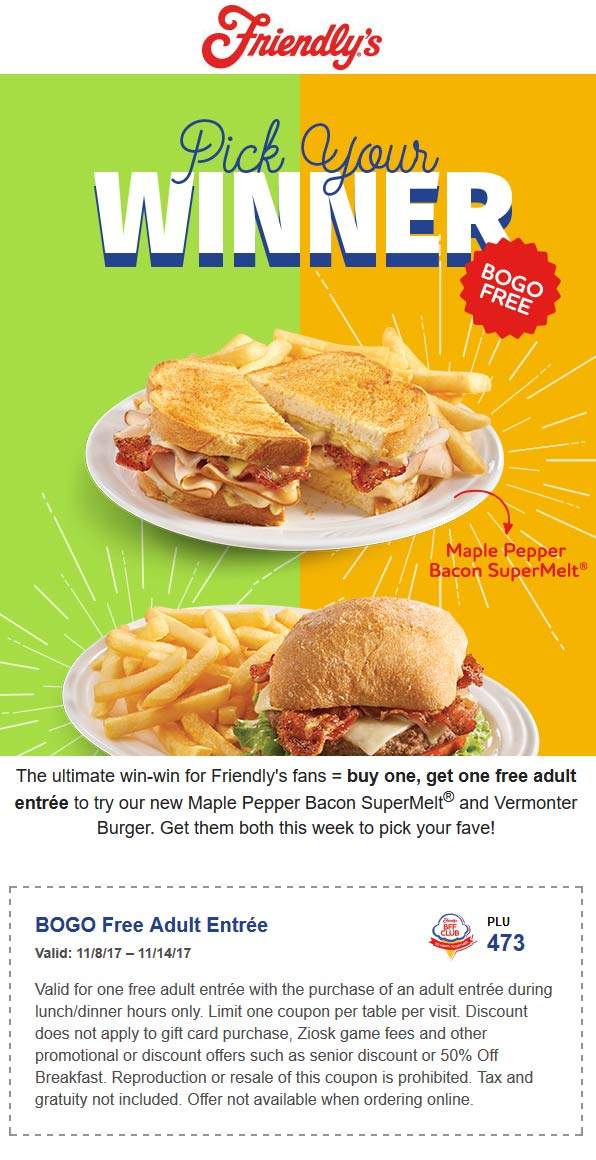The image is an advertisement for Friendly's restaurant. At the top center of the page, the Friendly's logo is prominently displayed in red text. Below the logo, the page is divided into two sections with different background colors: green on the left side and orange on the right. Centered on the page is the bold message, "Pick Your Winner," accompanied by a red circle containing the text, "BOGO FREE."

The advertisement features two enticing plates of food. The first plate showcases a delicious sandwich filled with bacon and various types of meat, layered between toasted bread, served alongside a generous portion of french fries. An arrow points to this plate, identifying the dish as the "Maple Pepper Bacon Super Melt."

Below this is a second plate on a white dish, also served with french fries. This sandwich includes bacon, lettuce, and tomatoes. The text beneath the plates reads: "The Ultimate Win-Win for Friendly's Fans. Buy one, get one free adult entree to try our new Maple Pepper Bacon Super Melt and Vermonter Burger. Get them both this week to pick your fave."

At the bottom of the page, there is a coupon offering a "BOGO FREE ADULT ENTREE," valid from November 8, 2017, to November 14, 2017. The terms and conditions specify that the coupon is valid for one free adult entree with the purchase of an adult entree, with a limit of one coupon per table per visit, among other details.